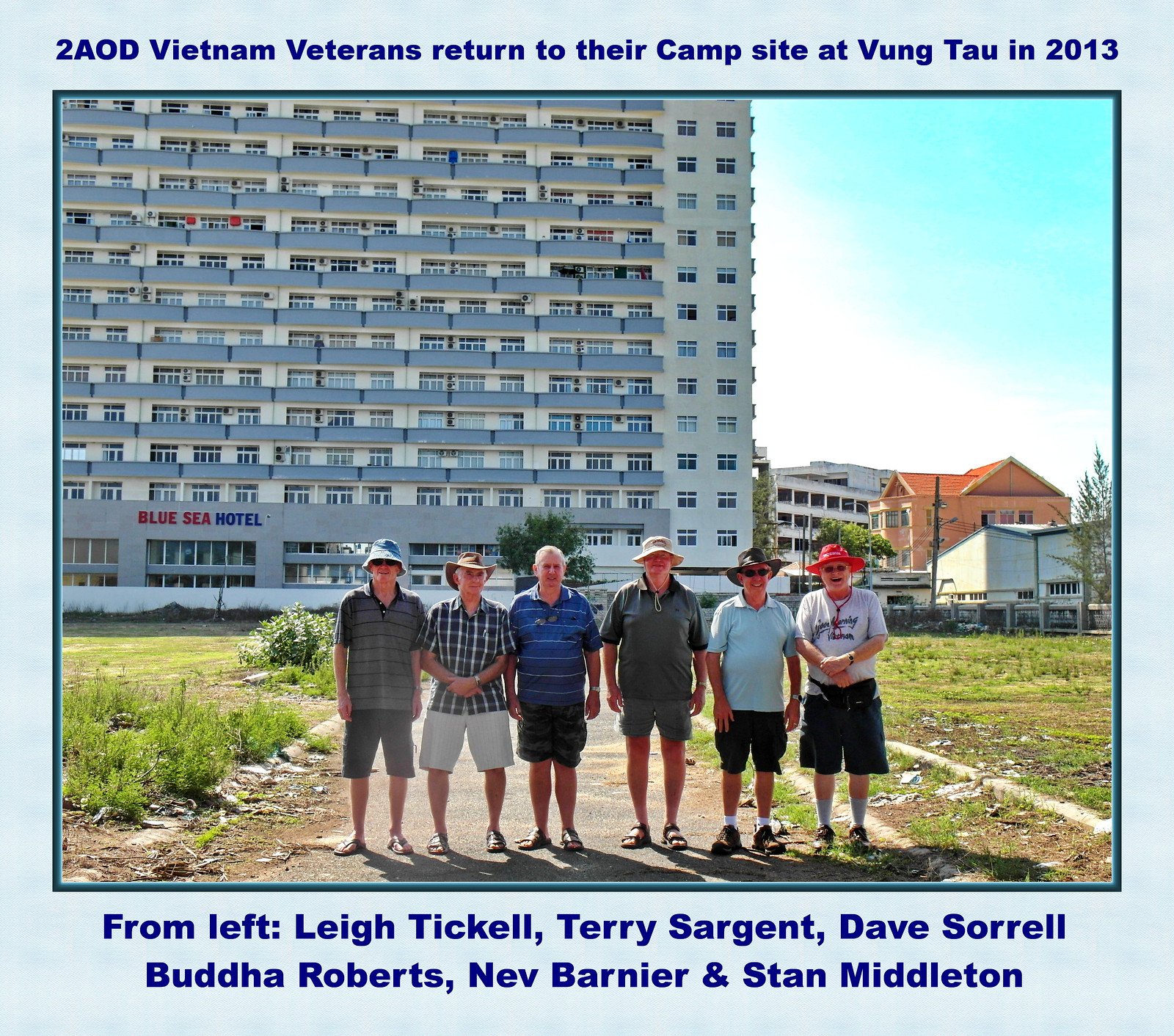In this outdoor photograph, six older men are lined up, smiling and posing for the camera in front of a tall, beige building with numerous balconies, which has a sign above the doors reading "Blue Sea Hotel." All wearing shorts and casual, warm-weather attire that includes sandals and wide-brim hats reminiscent of Australian styles—except for one man without a hat—they stand on a path surrounded by green bushes, dirt, and rocks. The setting appears to be an open, undeveloped lot. At the top of the image, a text caption reads, "Two AOD Vietnam veterans return to their campsite at Vung Tau, 2013." Below the photo, the men are identified from left to right as Leigh Tickell, Terry Sargent, Dave Sorrell, Buddha Roberts, Nev Barnier, and Stan Middleton. The sky above the buildings in the background is partly cloudy with shades of white and blue.